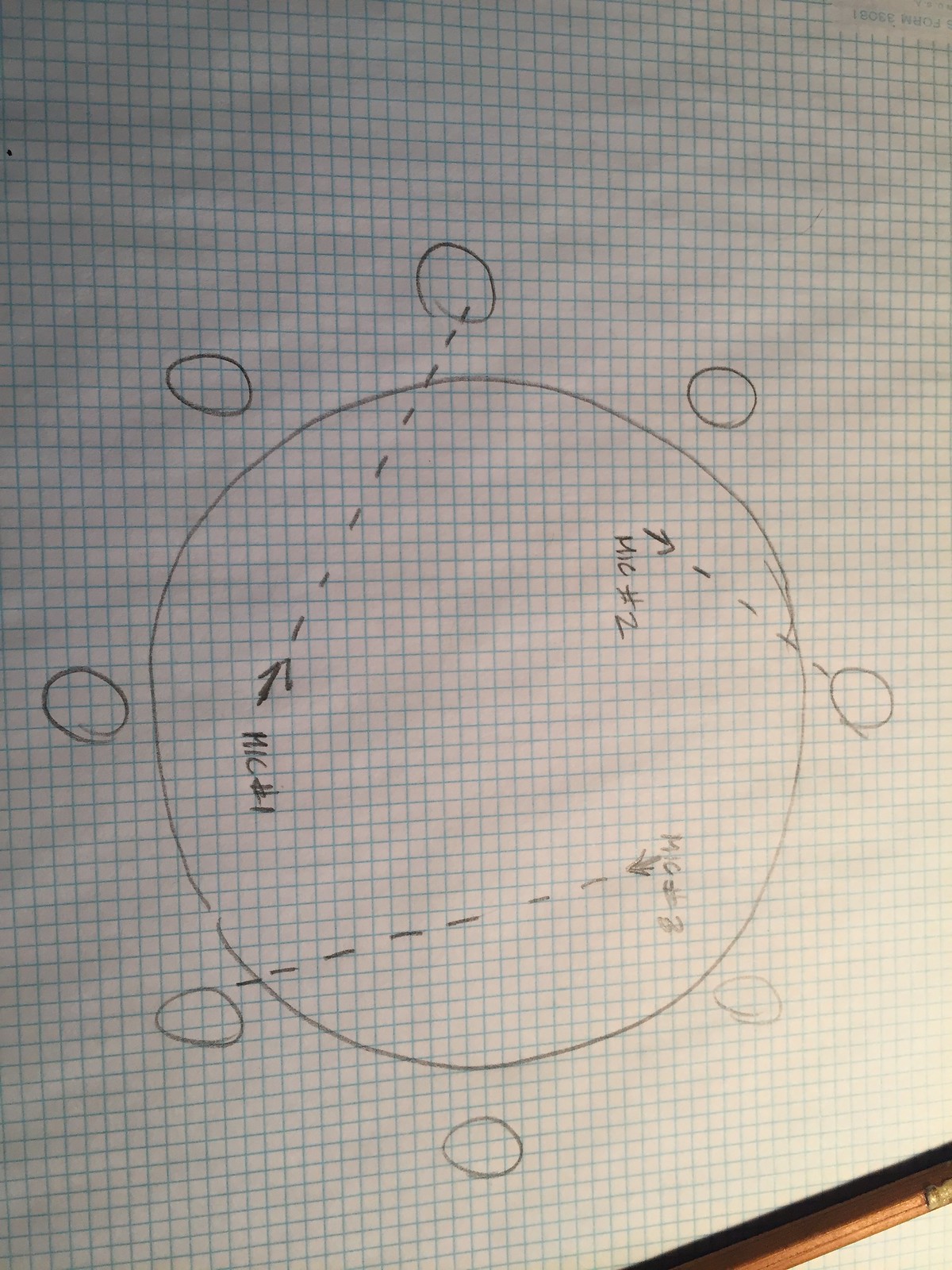The image depicts a piece of graph paper with blue lines, oriented sideways. In the bottom right-hand corner, there's a pencil resting on the paper, casting a shadow alongside it. On the graph paper, drawn in pencil, is a larger central circle with eight smaller circles surrounding it. These smaller circles, which are much smaller and appear hastily drawn, encompass the larger circle.

From the smaller circle positioned at what would be the nine o'clock position relative to the larger circle, a dashed line extends to the center of the large circle, annotated with the label "M.I.C. number one." Similarly, at the twelve o'clock position, another dashed line labeled "M.I.C. number two" leads to the smaller circle. Additionally, the smaller circle located at the five o'clock position is connected to the central large circle by a dashed line labeled "M.I.C. number three." The circles surrounding the central one are unevenly drawn, giving the diagram a rough and rushed appearance.